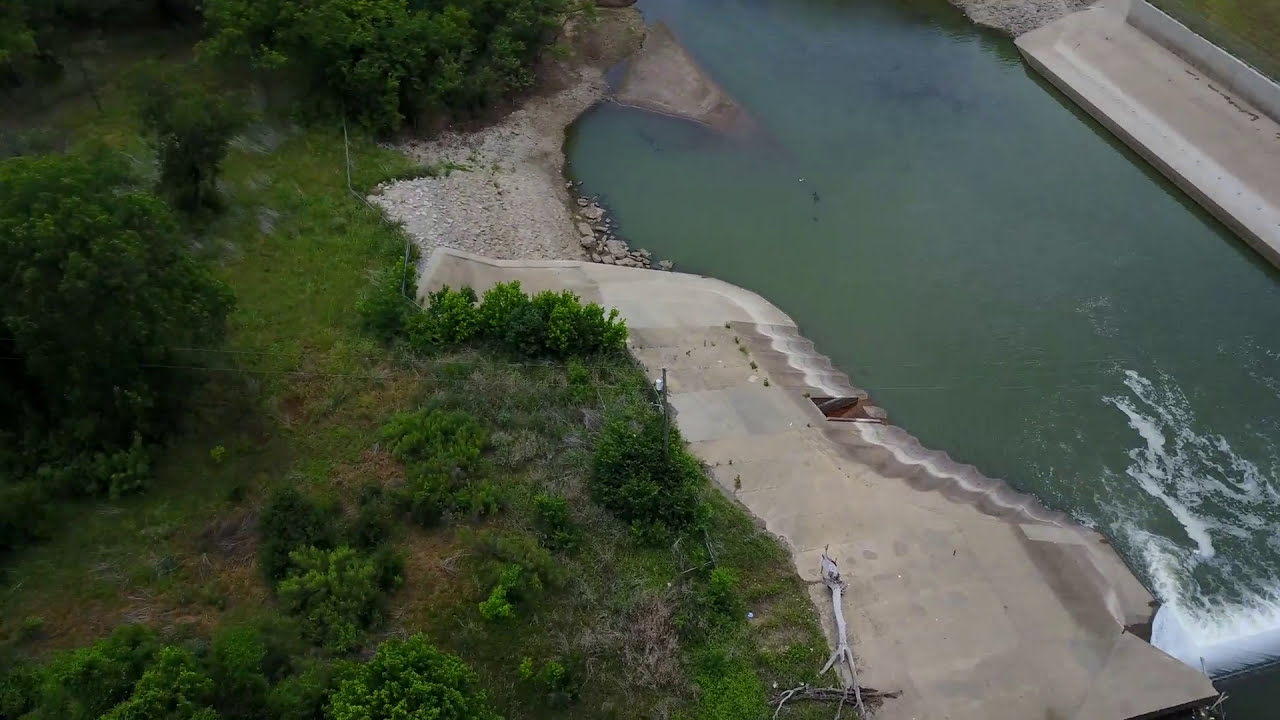The image depicts an aerial view of a waterway adjacent to a dam system, where the water has a greenish tint and forms a pond-like area. On either side of the water, concrete structures have been laid. The left side features a well-defined, square deck area, while the right side displays concrete ridges, possibly related to the dam functionality. There is a cutout within this structure, probably designed for water draw-off. At the bottom right, the water is churning and white, indicating more intense activity, suggesting the proximity of the dam. Surrounding the concrete boundary on the right side, there is a natural rocky shore leading to lush greenery, including grass, bushes, trees, and scattered branches.